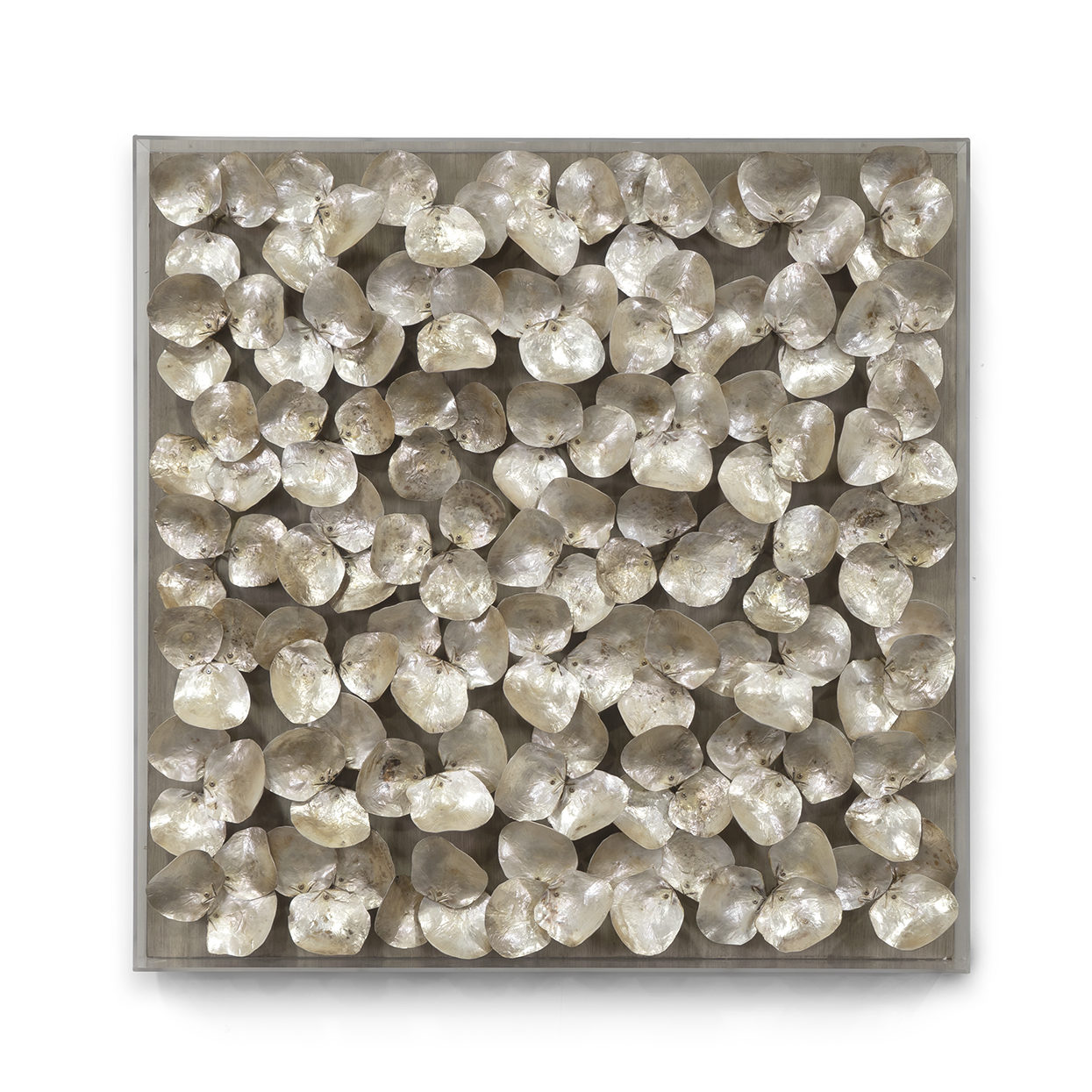This color photograph depicts a substantial collection of at least 200 stones, all predominantly round or oval-shaped, arranged meticulously within a square, three-foot by three-foot brown tray. The stones vary slightly in shape and size, with some being more rounded while others are longer and more oblong. They are primarily white or off-white, often exhibiting hints of light brown or small brown spots. The overall appearance suggests they could be uncut gems, possibly part of a jeweler's collection awaiting refinement. The stones’ subtle color variations and signs of wear add a natural and authentic aesthetic to the composition.